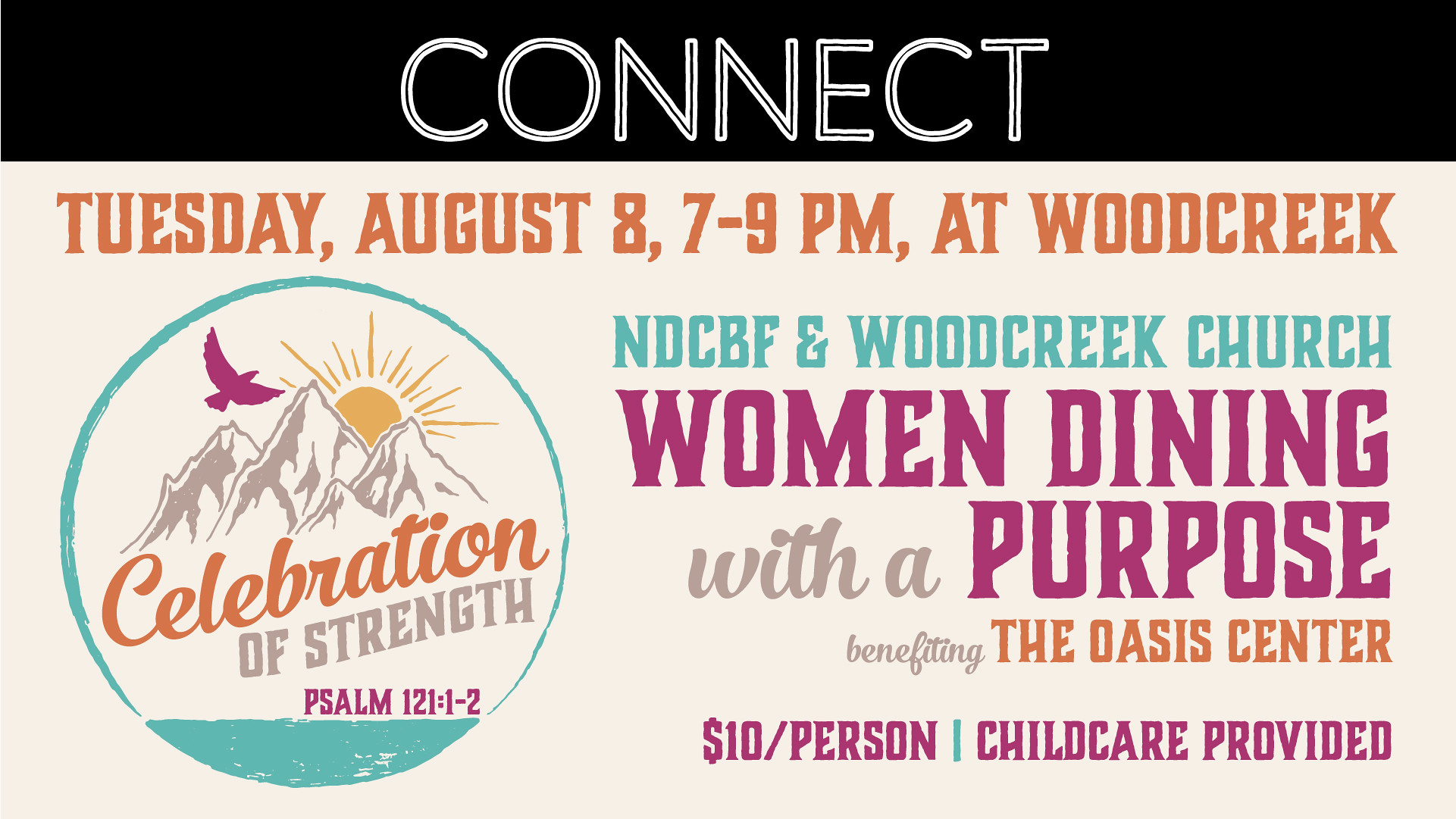This vibrant, modern advertisement features a prominent black header with the word "CONNECT" in bold white lettering. Below this header, on a white background, vital event details are written in various colors: "Tuesday, August 8th, 7 to 9 p.m. at Wood Creek" in eye-catching orange text. Beneath that, in a soothing aqua green, it reads "NDCBF and Wood Creek Church," followed by the event name in purple text: "Women Dining with a Purpose." The purpose of the event, benefiting the Oasis Center, is highlighted with "benefiting" in gray and "the Oasis Center" in orange. Additionally, in purple at the bottom, the advertisement notes, "$10 a person, childcare provided." On the left side, there is a circular logo with a green outline; it depicts a sun rising behind four mountain peaks with a bird flying overhead. The logo includes the text "Celebration of Strength," accompanied by the reference "Psalms 121:1-2."